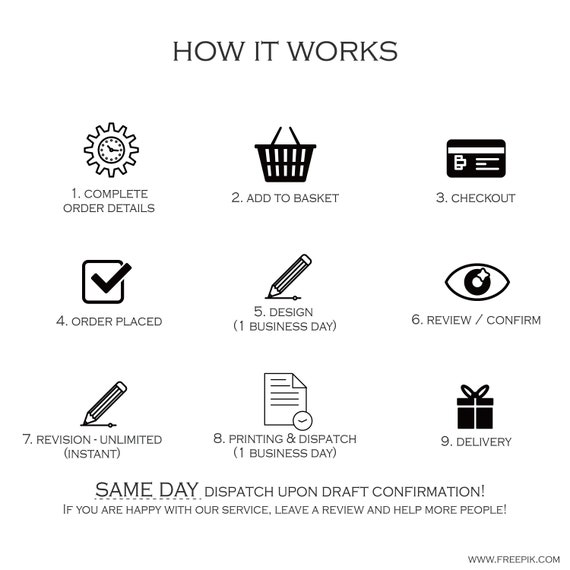The image is a black and white digital poster titled "How It Works." It consists of a 3x3 grid displaying nine sequential steps for a process, each illustrated with an icon. 

1. **Complete Order Details**: Represented by an analog wall clock inside a gear.
2. **Add to Basket**: Depicted by a shopping basket.
3. **Checkout**: Shown with a credit card icon.
4. **Order Placed**: Illustrated by a check mark in a box.
5. **Design (1 Business Day)**: Indicated with a pencil sketching a line.
6. **Review/Confirm**: Represented by an eye with a star on the pupil.
7. **Revise (Unlimited Instances)**: Depicted by another pencil icon.
8. **Printing and Dispatch (1 Business Day)**: Shown with a page featuring a folded top right corner.
9. **Delivery**: Illustrated by a gift box with a bow, with the note "Same day dispatch upon draft confirmation."

At the bottom, the poster urges viewers to leave a review if satisfied with the service, with the web address www.freepic.com placed in the bottom right corner.